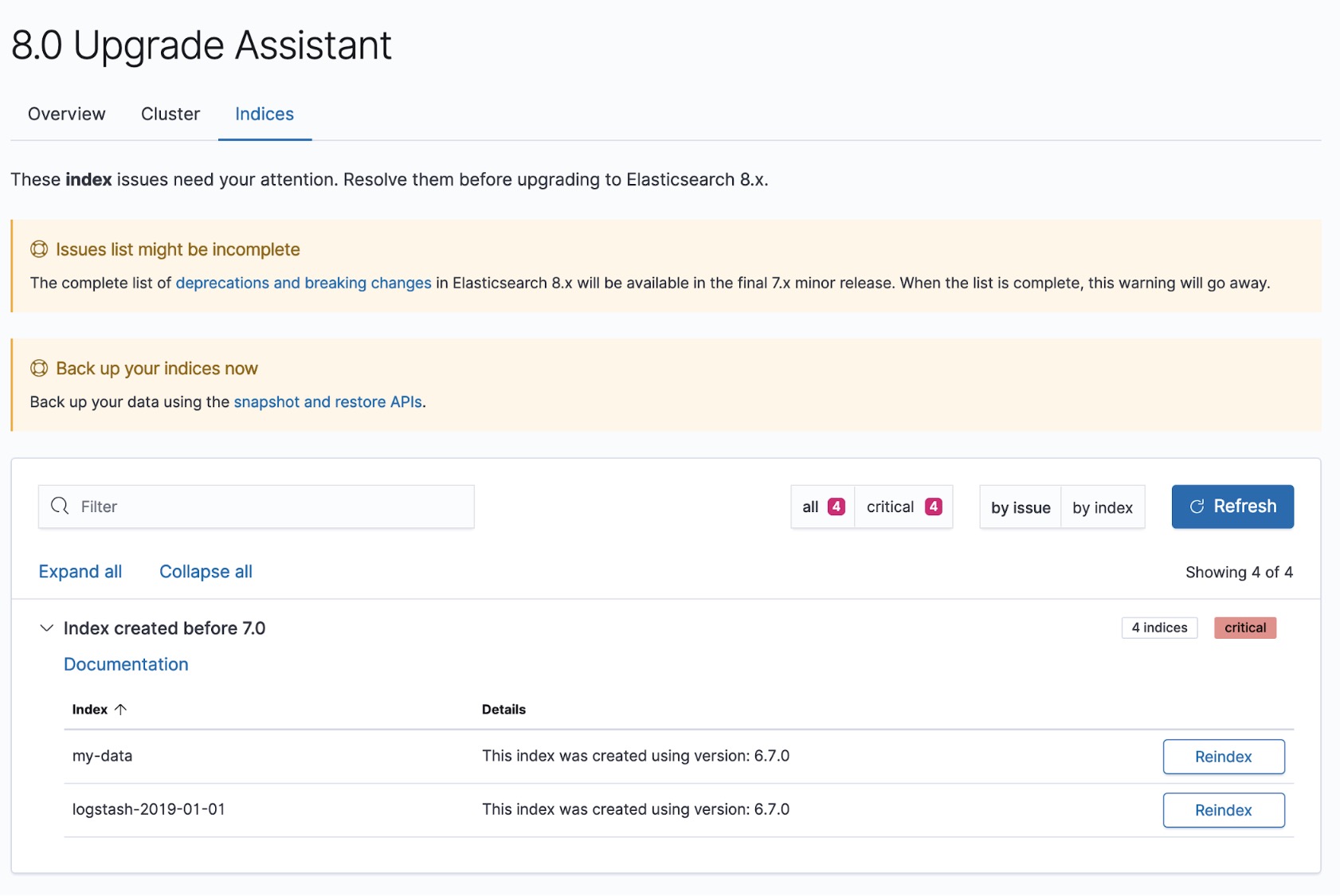In this detailed image of the "8.0 Upgrade Assistant" interface, the top prominently displays the title "8.0 Upgrade Assistant" in large black font. Directly beneath this, there are three tabs labeled "Overview," "Cluster," and "Indices." Below these tabs, a thin grey line separates them from the next section, which features a crucial alert stating, "These index issues need your attention. Resolve them before upgrading to Elasticsearch 8.x."

A notable yellow tab warns, "Issues list might be incomplete. The complete list of deprecations and breaking changes in Elasticsearch 8.x will be available in the final 7.x minor release. When the list is complete this warning will go away." Adjacent to this, another important reminder reads, "Backup your indices now. Backup your data using the snapshot and restore APIs."

Further down, there is a search bar labeled "Filter" with an accompanying magnifying glass icon for ease of searching. Under this, options in blue font allow users to "Expand All" and "Collapse All" items. The interface also features segments categorized as "All" and "Critical by issue by index," with a refresh button highlighted in blue for updating any changes.

The background of the page is predominantly white, providing a clean and organized look. Scattered across the interface are the words "Documentation" in blue, indicating additional resources. Notably, there are two prominent buttons labeled "Re-index," guiding users towards this crucial action.